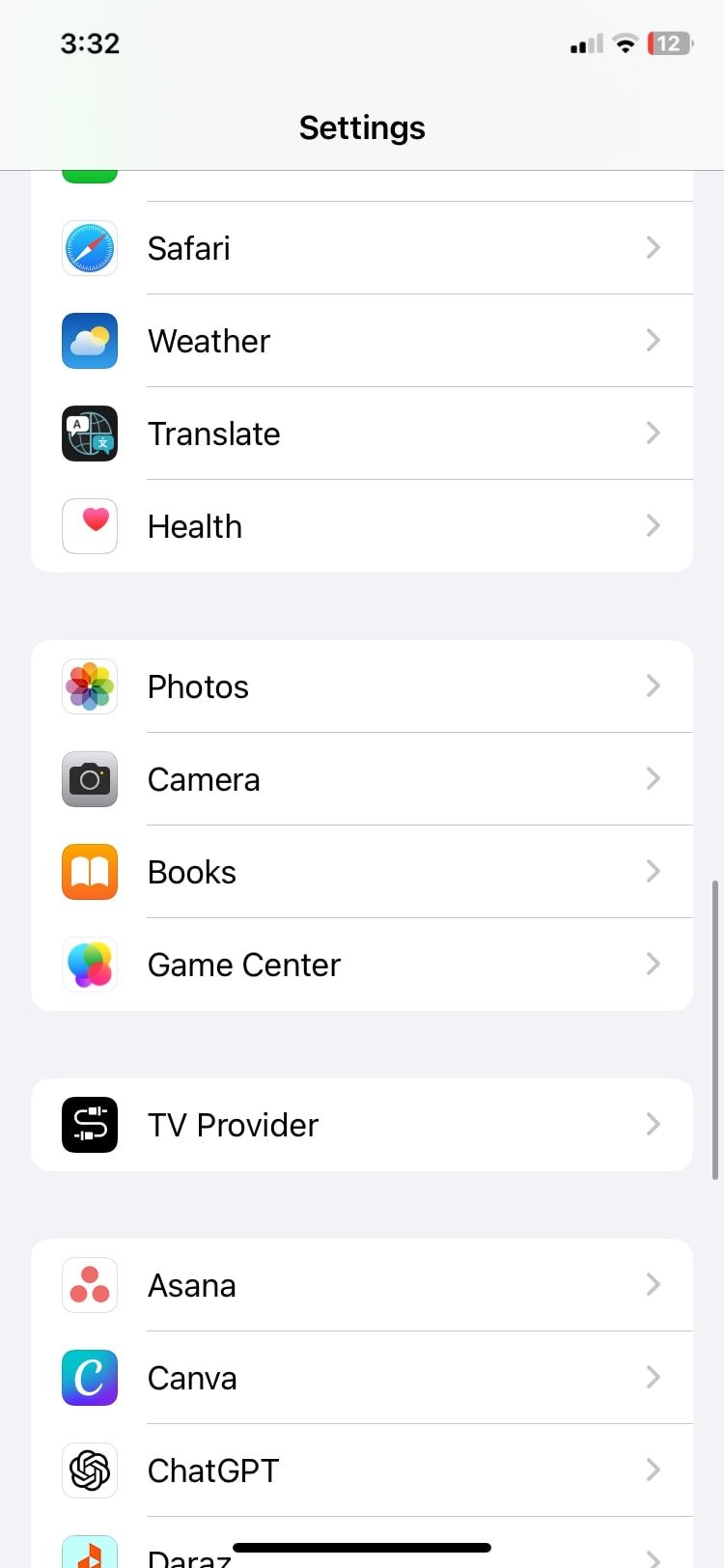**Descriptive Caption:**

The screenshot taken from a smartphone shows a light gray background. The status bar at the top of the screen indicates the time is 3:32 PM, and the battery level is critically low at just 12%. Dominating the center of the screen is the title "Settings," displayed in gray. Below the title, a series of neatly arranged, white-background rectangular icons and items are listed.

The first row features various icons for typical apps: "Safari" (the web browser), "Weather," "Translate," and "Health." The "Health" icon stands out with its design, a white square featuring a red heart in the center.

As we move down the list, we see icons for "Photos," "Camera," "Books," "Game Center," and "TV Provider." Further down, the apps "Asana" and "Canva" are listed, with the "Canva" icon designed as a blue and green square with a white 'C.' Finally, at the bottom of the list, the "ChatGPT" app is displayed.